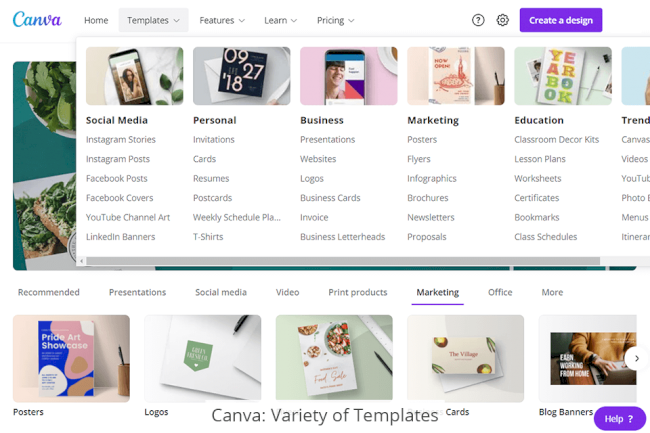The image displays Canva's homepage, characterized by its distinctive blue and purple color scheme. In the upper left corner, the Canva logo is prominently featured. The main navigation bar, filled with multiple tabs, includes the following options: Home, Templates, Features, Learn, and Pricing. 

The Templates tab is highlighted in gray, with a drop-down menu showcasing a variety of categories and corresponding sub-options. Within this menu, the categories and their options are outlined as follows:

1. **Social Media**:
   - Instagram Stories
   - Instagram Posts
   - Facebook Posts
   - Facebook Covers
   - YouTube Channel Art
   - LinkedIn Banners

2. **Personal**:
   - Invitations
   - Cards
   - Resumes
   - Postcards
   - Weekly Schedule (partially cut off)
   - T-Shirts

3. **Business**:
   - Presentations
   - Websites
   - Logos
   - Business Cards
   - Invoices
   - Business Letterheads

4. **Marketing**:
   - Posters
   - Flyers
   - Infographics
   - Brochures
   - Newsletters
   - Proposals

Below this drop-down menu, the homepage features a series of recommended sections, including Presentations, Social Media, Video, Print Products, Marketing, Office, and More. Among these, the Marketing section is underlined, drawing attention to various thumbnail previews of different projects that can be created using Canva's tools.